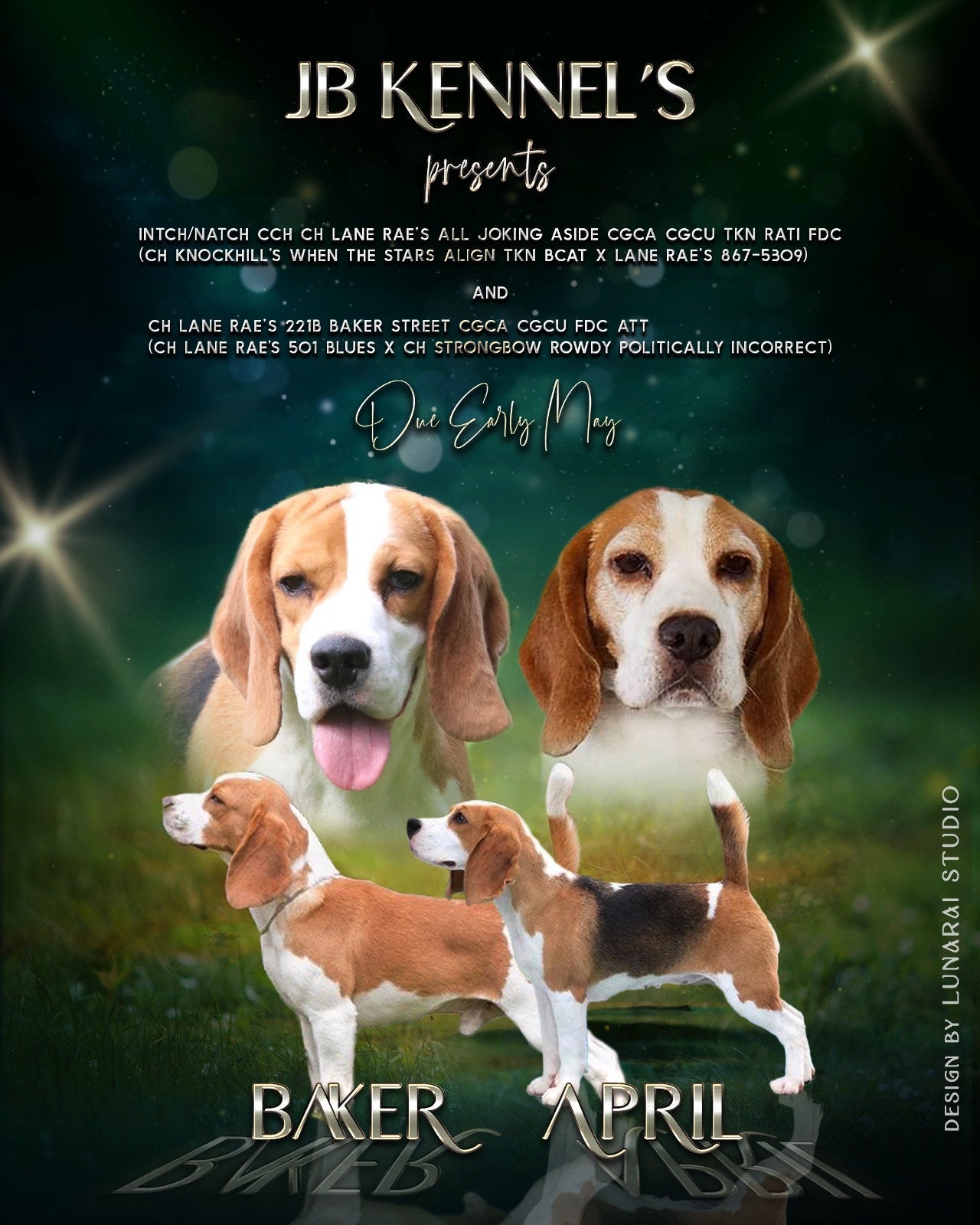This poster ad, set against a dark green background with light green grass at the bottom and illuminated by lens flares and star-like dots, prominently features two beagles presented by JB Kennels. At the top, in luxurious gold and silver font, the text "JB Kennels Presents" is displayed, followed by an array of abbreviations indicating the dogs' pedigrees and titles, including champions such as "CCH CH Lane Rays All Joking Aside CG CA CG, CH Knock Hills When the Stars Align", and "CH Lane Rays 221B Baker Street CG GA GCG CU FTC ATT Champion Lane Rays 501 Blues ex-Champion Strongbow Rowdy Politically Incorrect."

Centrally placed in the poster are two beagles, each displayed both facing forward and in profile. The beagle on the left, named Baker, is white and tan, depicted happily with its tongue out. This dog is also shown in profile facing left, under the name "Baker" in silver letters. The dog on the right, named April, is similar in coloration but with additional black markings. April appears older with some graying around the eyes and is also shown in profile facing left, with the name "April" displayed underneath in silver letters. Both dogs are set against the green, star-studded background, which gives the appearance of their names shining on the floor. This detailed and luxurious ad captures the distinguished nature of these beagle champions, highlighting their esteemed heritage and inviting spectators to witness their showcasing.